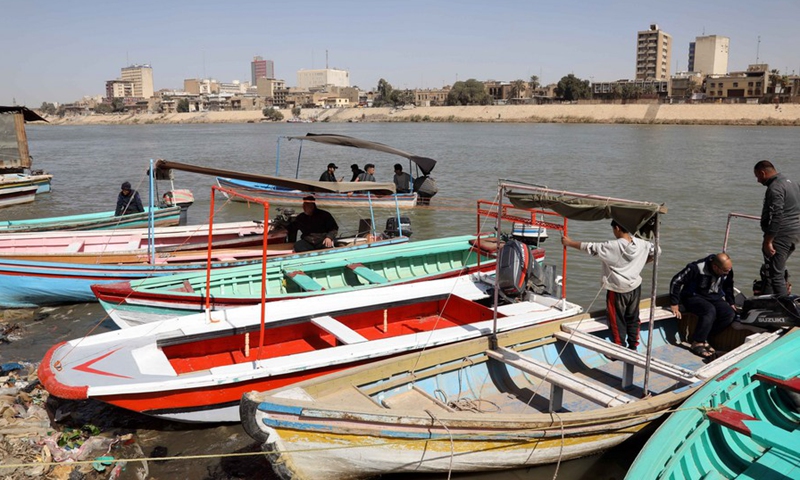The image captures a bustling marina filled with a variety of wooden boats in an array of colors including pale tan, mint green, red and white, and pale pink. Within the marina, five to six boats are visible, most of them securely moored, yet one boat is beginning to venture out into the expansive water. The vibrancy of the scene is further accentuated by the presence of men of Middle Eastern or Indian descent on board these boats, engaged in various activities. The water exhibits a grayish hue, which is echoed by the overcast sky above—a sky that suggests haze, possibly from pollution, rather than clouds. The backdrop reveals a sprawling cityscape with towering skyscrapers, adding an urban contrast to the otherwise serene maritime setting. The beach lining the water’s edge is a pristine white sand, while a cluster of dark green plants punctuates the scene. The lush greenery and the overall ambient temperature hint that this moment is captured during the summer season.